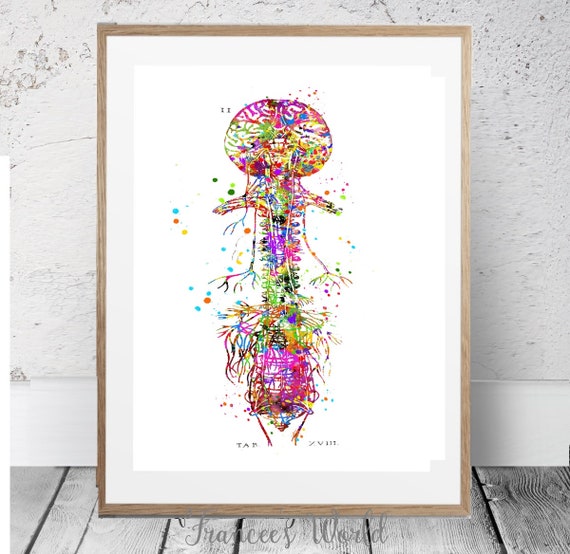The image showcases a vibrant, colorful painting placed at the center against a white stucco wall. The painting, set in a light brown, washed-out wooden frame, leans against the wall, which features some visible cracks and dots. Below the wall, a board connects it to a floor made of light gray, vertically laid, wooden planks.

The artwork itself is an abstract, multi-colored depiction of a brain and spinal column. It starts with a brain-like structure at the top, distinguished by its lobe-like forms, and continues with a spine-like body towards the bottom. Surrounding the central shapes are numerous colorful dots in shades of pink, blue, green, yellow, white, and fuchsia, adding to the painting's visual complexity.

In addition, there’s a light blue mat around the artwork enhancing its presentation. At the bottom center of the image, inscribed in light grey, is the text "Francine's World."